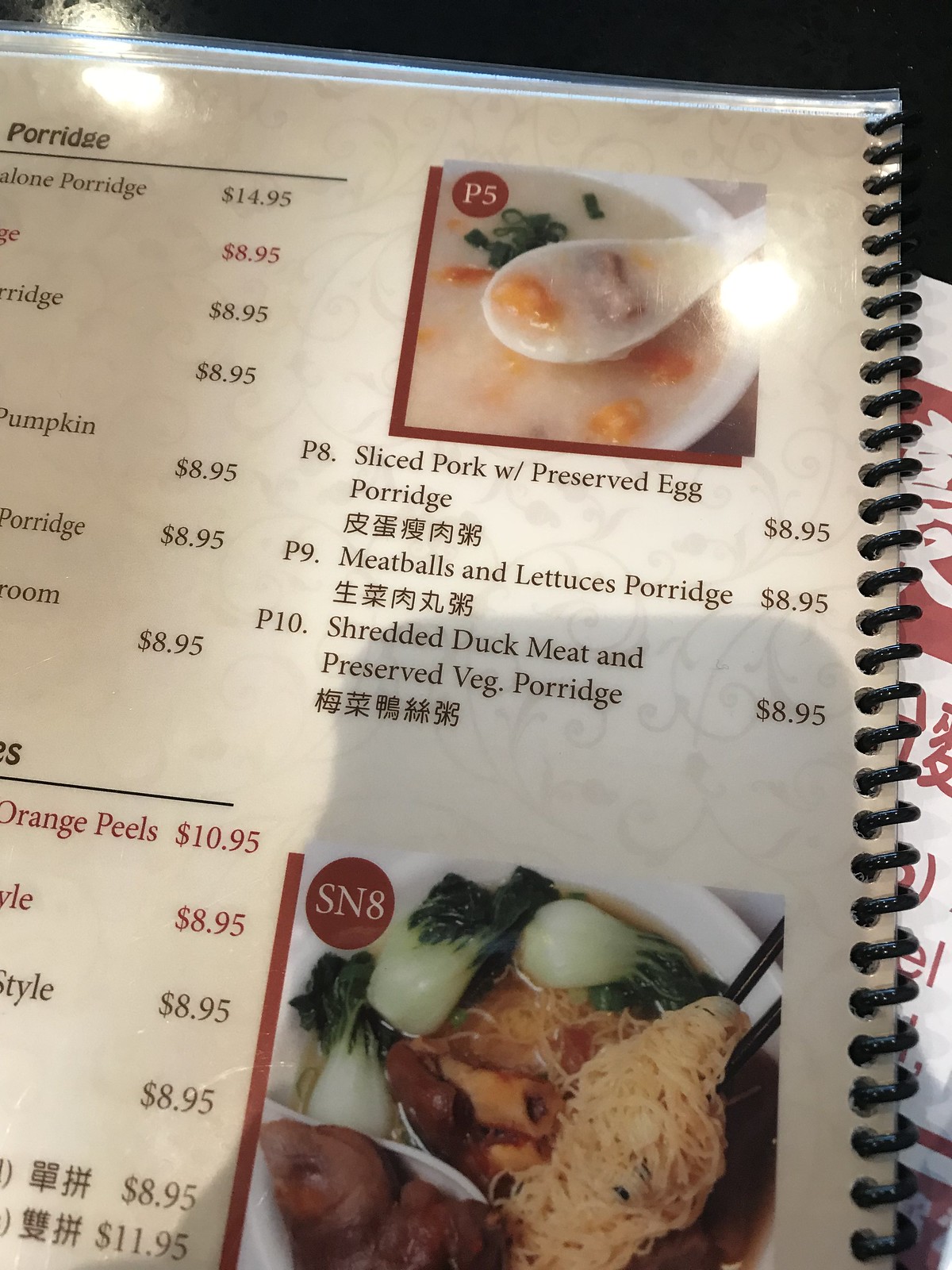The image features a partially cropped, spiral-bound restaurant menu, captured with a regular camera. At the top of the visible page, there's a photograph marked with a "PS" in the corner, depicting a bowl of soup. A spoon is emerging from the soup, holding pieces of chicken and carrot. Below the image, the menu lists the following items:

- Sliced Pork with Preserved Egg Porridge - $8.95
- Meatballs and Lettuces Porridge - $8.95
- Shredded Duck Meat and Preserved Veggie Porridge - $8.95

Towards the bottom of the menu, there is another image showcasing a mix of onions, possible potatoes, and shredded cabbage with a peachish hue.

On the left side of the menu page, additional items and prices can be glimpsed:
- Various Porridge options priced at $14.95, $8.95, $8.95, $8.95, $8.95, $8.95, and $8.95
- Orange Peels - $10.95
- A dish labeled "Style" - $8.95
- Additional items priced at $8.95, $8.95, and $11.95

Despite the cropped portions, the detailed items and prices provide a glimpse into the offerings of the menu.